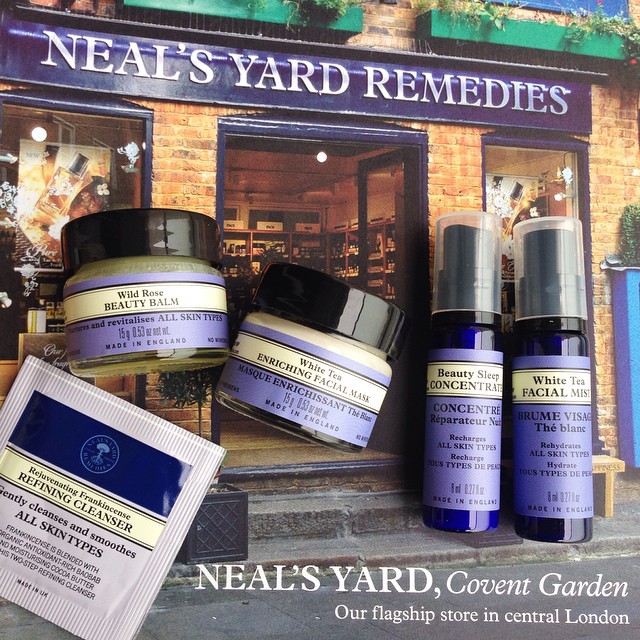The image features a detailed photograph of the storefront for Neal's Yard Remedies, distinguished by its prominent blue sign with white text reading "Neal's Yard Remedies." The storefront is located in an outdoor setting, with a stone or asphalt street and stairs leading up to the entrance, indicating it's a daytime scene. At the bottom right corner of the photo, there is additional text that reads, "Neal's Yard, Covent Garden, our flagship store in central London." In front of the photograph are five beauty products positioned centrally. On the left is a small packet labeled "Rejuvenating Frankincense Refining Cleanser," described as gently cleansing and smoothing all skin types. Next, there are two jars: the one on the left is labeled "Wild Rose Beauty Balm," and the one on the right is "White Tea Enriching Facial Mask." The arrangement of these products and the photo creates a vivid advertisement showcasing Neal's Yard Remedies' beauty offerings, set against the backdrop of their flagship store. The products come in various colors, including blue, green, brown, purple, yellow, orange, and gray.